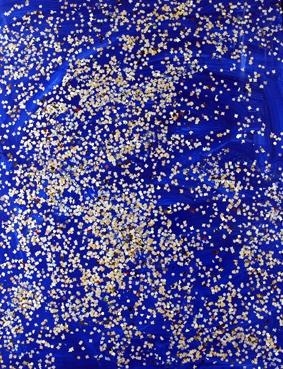This image is a tall rectangular design featuring a vibrant royal blue background interspersed with darker navy blue shades, creating a textured appearance with subtle striations and shadows. Randomly scattered across this blue expanse are numerous tiny white flecks and beads, with colors ranging from pure white to tan gold and even some black. These beads are densely concentrated in certain areas, most notably in the middle left section, where they form a thick cluster, and then dispersed more sporadically towards the upper right, allowing for broader visibility of the intricate blue background. The image overall presents a dynamic, almost abstract pattern that is both visually captivating and texturally rich.